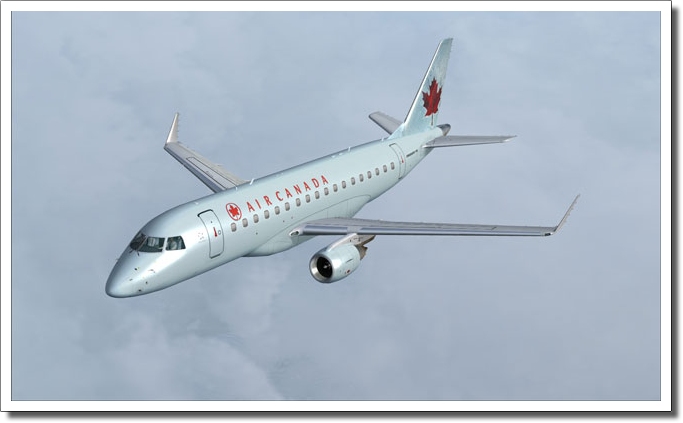This detailed depiction showcases a silver-colored Air Canada commercial aircraft, prominently displaying the iconic red maple leaf logo. The image captures the plane from a front-right side profile, soaring above misty gray clouds that lack sharp detail. The aircraft's body is a silvery blue hue, with the wings appearing more gray. The branding is clearly visible with "Air Canada" printed in red above the passenger windows, accompanied by the red maple leaf encircled in a ring. The same distinctive maple leaf insignia adorns the tail fin. This jet-engine plane is reminiscent of models from the 1980s, and although you can see pilots through the cockpit windows, there's a sense of isolation against the overcast sky.